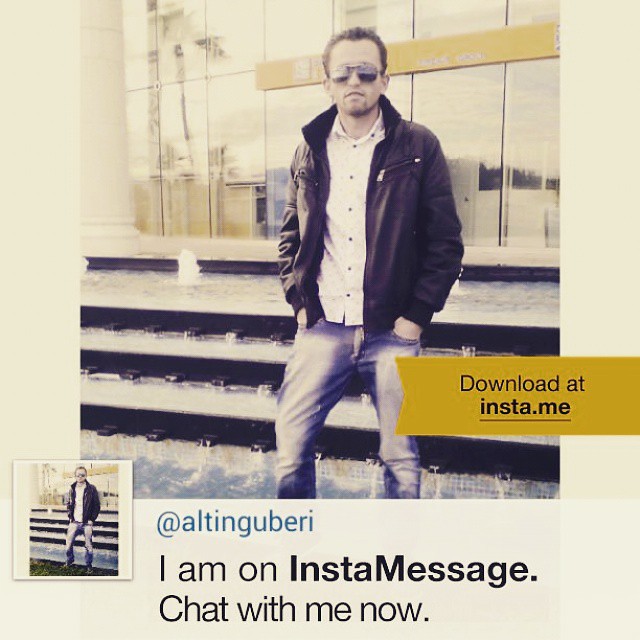In this image, a man in his late 20s to early 30s is standing confidently in front of a warehouse entrance or possibly near some railroad tracks. He has short brown hair and is wearing mirrored aviator sunglasses while looking straight into the camera. He is dressed in a black leather jacket that resembles a police or union work coat, a white button-down collared shirt, and faded blue Levi denim jeans. The backdrop includes a staircase leading to a building with visible windows, palm trees reflected, suggesting a warm climate, likely Florida or California.

The photo appears to be part of a promotional handout or an album cover, presented on an off-white background. Emphasized details include a yellow or gold banner towards the bottom right, stating "Download at insta.me," which is underlined. Below the primary image, there is a smaller inset of the same picture at the bottom left corner. Adjacent to this inset, it reads "at altinguberi" in blue text, followed by the black text, "I am on InstaMessage. Chat with me now." This layout indicates that the man is likely a music artist promoting his presence on InstaMessage to engage with his audience.